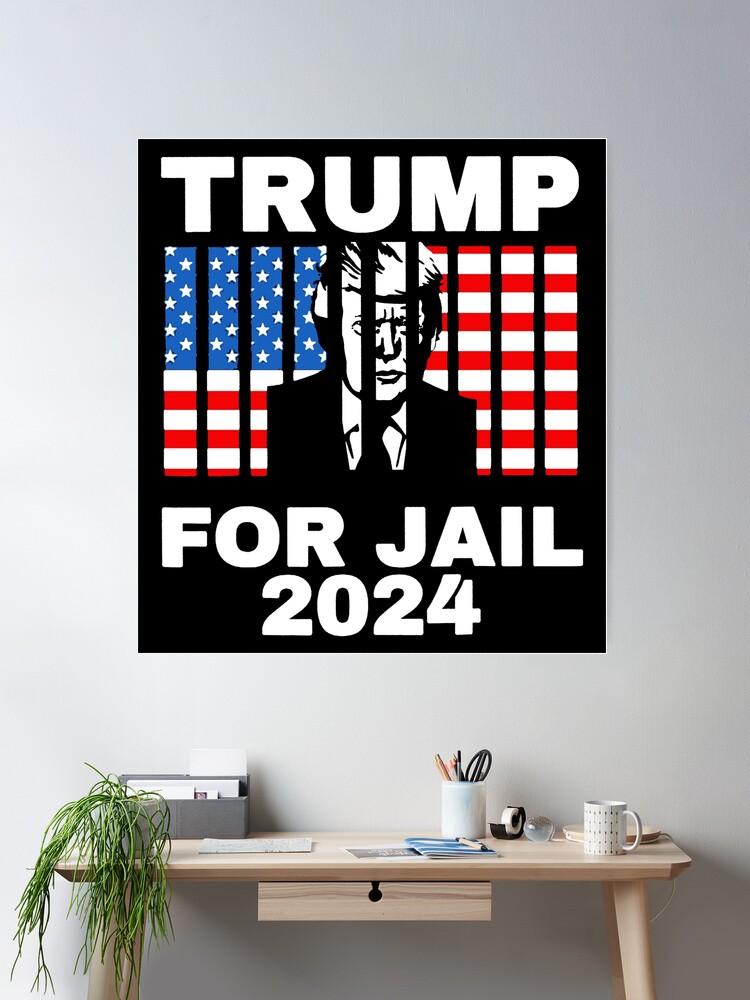The image showcases a minimalistic setup with a striking, computer-generated poster as the focal point. The poster is affixed to a pristine white wall and features a black background with bold white text at the top reading "TRUMP" and at the bottom "FOR JAIL 2024." In the center, it depicts a black-and-white image of Donald Trump set against an American flag with black vertical bars resembling jail bars. Below this arresting poster, a compact light wood-colored desk is neatly arranged. On the right side of the desk rests a small white desk lamp, angled over the workspace. In front of the lamp, a white coffee mug can be seen. Moving leftward, there is a roll of tape beside another white container holding pens and pencils. Scattered brochures and a subtle, small green hanging plant cascading over the left edge complete the scene. The desk also features a drawer underneath, providing additional storage space. The overall composition exudes a blend of simplicity and stark political commentary.